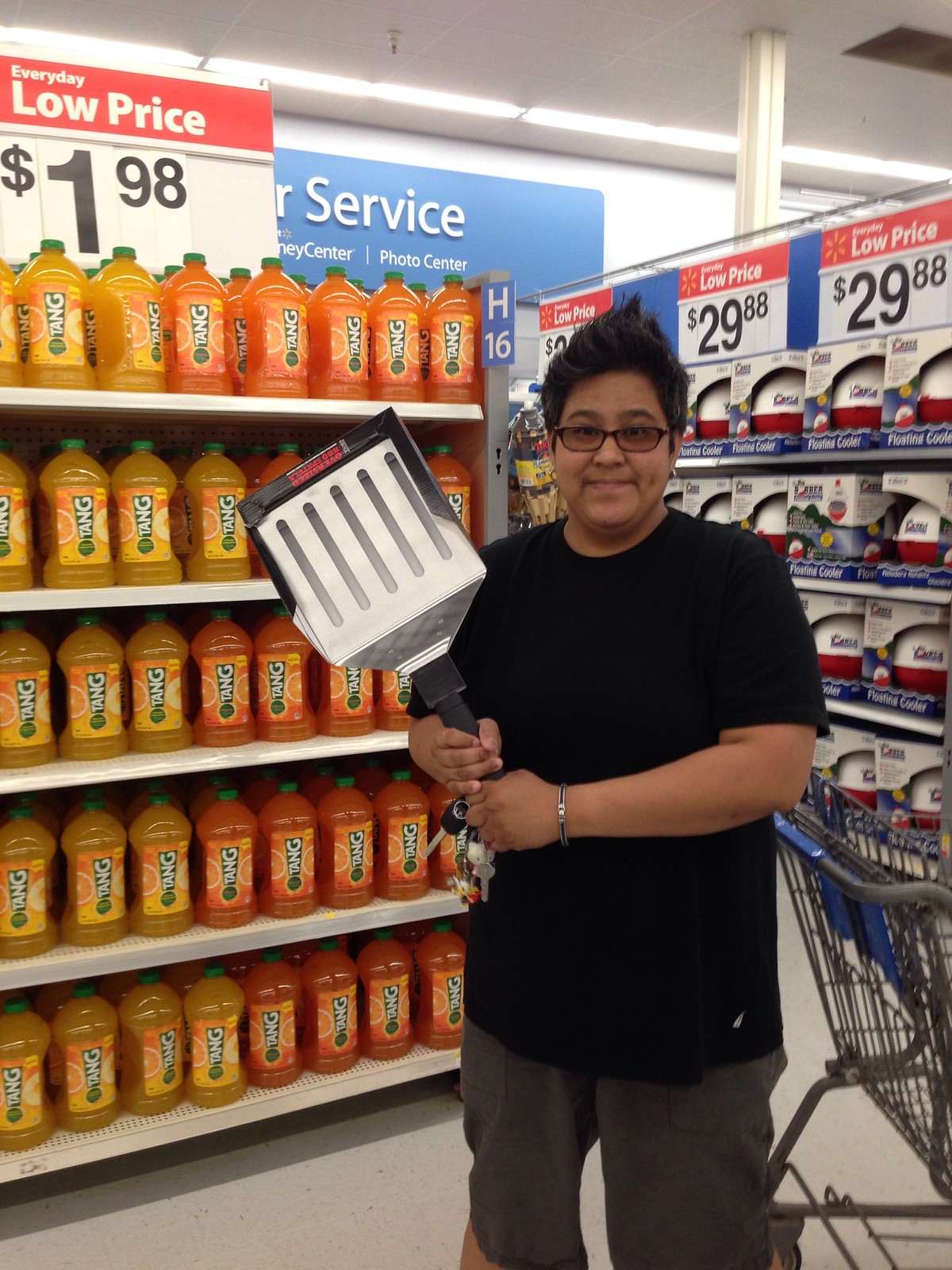This is a color photograph of a person standing inside a Walmart store. The individual, with short, poofy black hair and glasses, is wearing a black t-shirt and gray shorts. In their right hand, they are holding a large metal object that resembles a giant spatula with a black handle, and they also have keys. To the left of this person is a shopping cart. The store features white walls and is brightly lit by fluorescent lights. Behind the person, there is a display with bottles of orange soda labeled "Tang" and a sign that reads "Everyday Low Price $1.98." Additionally, there is another sign displaying "Floating Cooler $29.88." The floor appears to be white, and the overall scene captures a typical supermarket setting with neatly stacked products and clear pricing signage.